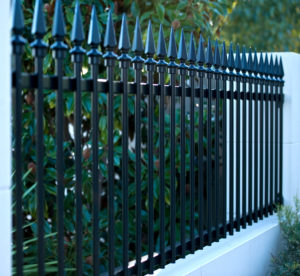The image depicts a close-up view of a black wrought iron fence with sharply pointed spikes atop each post, designed to enhance security. The fence is mounted on a concrete base and is attached to a wall on its right side. Behind the fence, a variety of green shrubbery and trees provide a natural backdrop. The scene is framed by green grass at the bottom right of the picture and extends upward, revealing additional greenery. There are no textual elements in the photograph. The fence, though sturdy, appears relatively short and would not be very effective at preventing intrusion despite its spiked design. The overall color palette in the image consists mainly of green, black, and white.